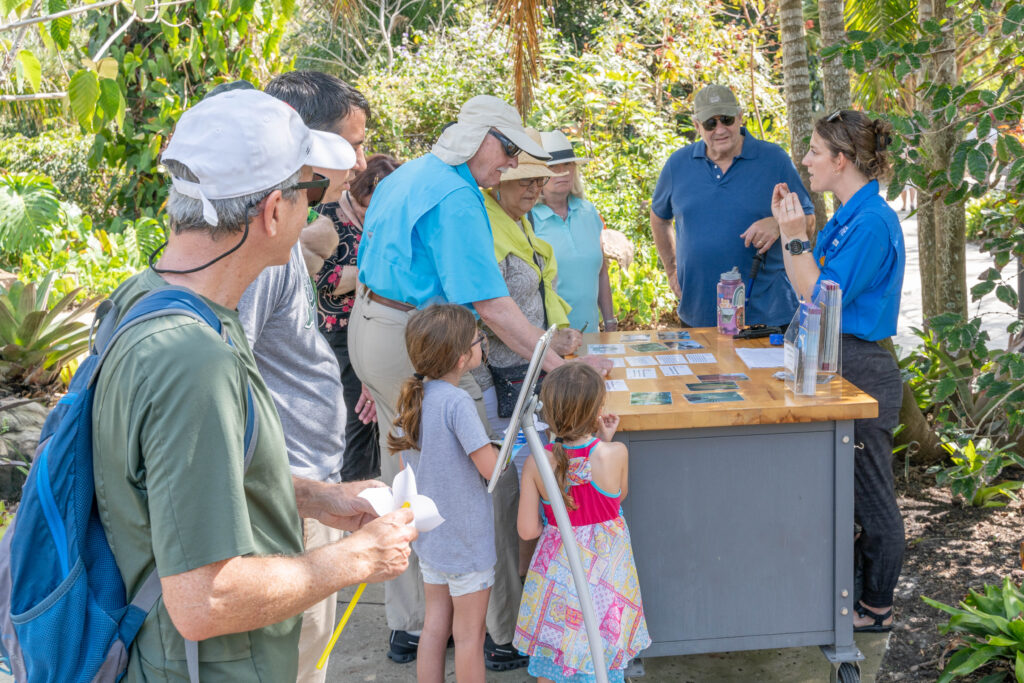In an outdoor setting surrounded by lush tropical foliage and water glimpsed behind the trees, a group of eight adults and two children gather around a wooden-topped, grey-sided table on wheels. The table is set up on a cement surface and is scattered with various postcards or cards. The focus of the group is a woman standing to the right behind the table, wearing a blue button-up shirt, black pants, black sandals, and a black watch. Her brown hair is swept back in a bun with sunglasses perched on top. The warm weather is evident as most people are in short-sleeved shirts, many sporting sunglasses and baseball hats. The woman appears to be explaining something to the attentive crowd, possibly as a tour guide or zookeeper, while a man in a dark blue shirt next to her engages in a conversation with her.